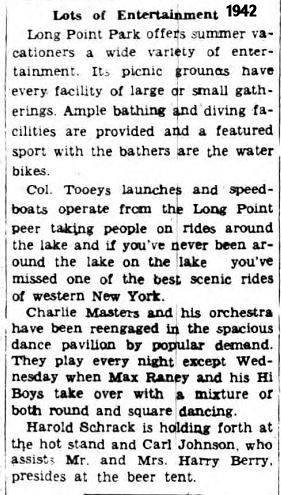The image appears to be a low-resolution scan of an old newspaper article from 1942, marred by significant JPEG artifacting. The headline reads, "Lots of Entertainment 1942," and the text spotlights Long Point Park as a prime summer destination offering a plethora of activities. The park's picnic grounds accommodate both large and small gatherings. It boasts ample bathing and diving facilities, with water biking being a particularly popular activity. Special attractions include Colonel Tooey’s launches and speedboats, providing scenic tours of Western New York from Long Point Pier. Additionally, the venue features live music; Charlie Masters and his orchestra play nightly in the spacious Dance Pavilion, except on Wednesdays when Max Rainey and his High Boys perform a mix of round and square dancing. Harold Schreck manages the hot stand, while Carl Johnson helps Mr. and Mrs. Harry Berry at the beer tent. The overall appearance suggests this is a historic and well-loved location for summer fun.